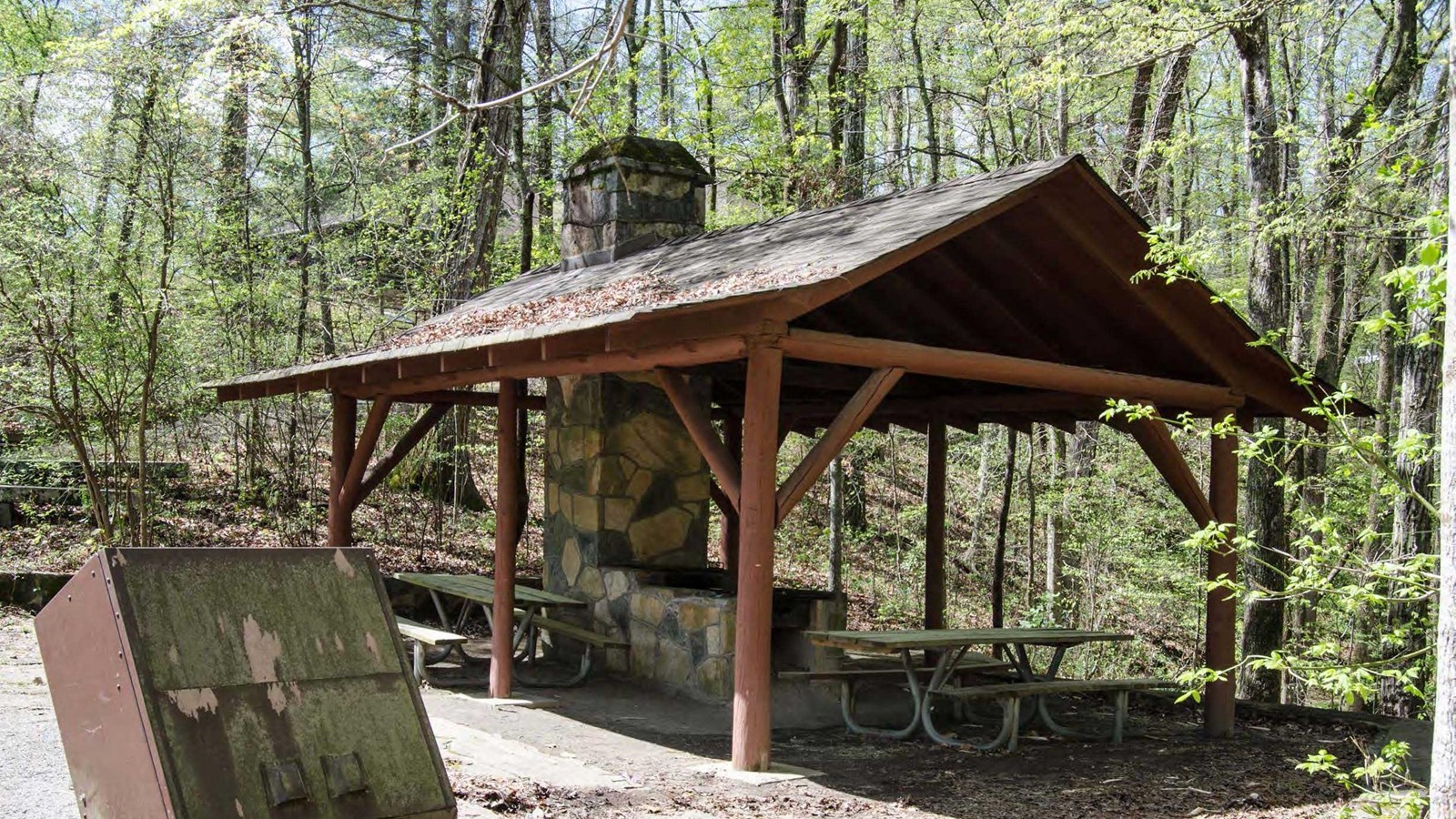This photograph showcases a weathered and somewhat dilapidated gazebo set within a hilly forest landscape. The structure, appearing slightly off-center to the right, is constructed from cylindrical wooden posts that support an A-shaped roof made of wood. Underneath the open roof, the gazebo features a concrete floor, two green weathered benches with metal legs, and a prominent fireplace. The fireplace, crafted from tan, black, and brown stones, has an oblong fire pit and a chimney that extends through the back of the roof. There is also a brown metal box situated near the structure, and a deteriorated metal sign, possibly an old map, indicating a hiking trail entry point. This gazebo, lacking walls, serves as a rustic eating or resting area, equipped with picnic benches and surrounded by scenic wooded trails.